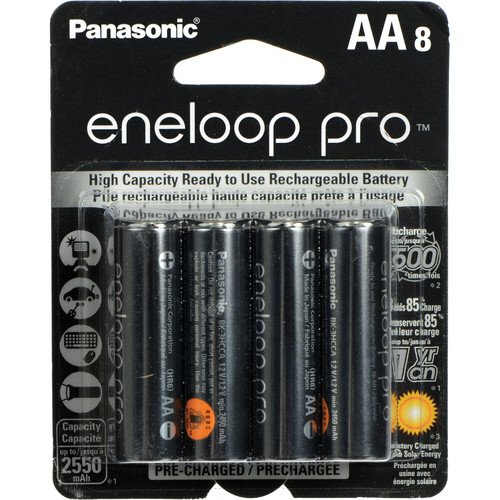This image features a meticulously presented package of Panasonic Eneloop Pro AA batteries, an 8-pack, ideal for demanding devices. The packaging clearly identifies the brand as Panasonic and the model as Eneloop Pro. Each AA battery boasts a high capacity of 2,550 mAh, arriving pre-charged and ready for immediate use. These rechargeable batteries can be recharged up to 500 times, showcasing impressive sustainability by retaining up to 85% of their charge even after one year of non-use. 

The packaging underscores the batteries' suitability for high-drain devices such as cameras, flashlights, and game controllers, emphasizing their dependable performance and longevity. Notably, the transparent plastic casing offers an unobstructed view of the neatly arranged batteries, enhancing confidence in the product’s quality. The sleek black and silver design, along with prominent branding, contributes to a professional and premium appearance, elevating the overall aesthetic appeal. This thoughtful presentation reflects a blend of functionality and sophisticated style, making the Panasonic Eneloop Pro batteries a preferred choice for those seeking both performance and elegance.